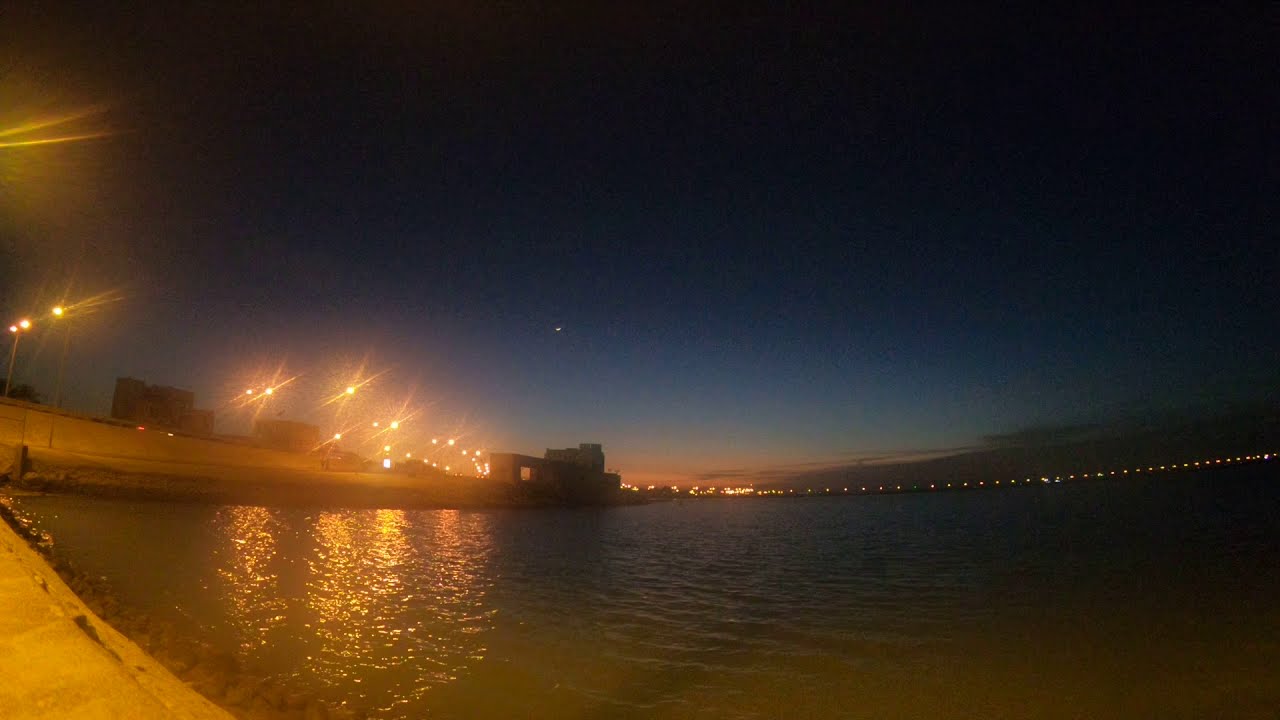A picturesque nighttime scene captures the calm of a bay area, illuminated by a string of twinkling yellowish lights lining the shoreline. On the left side of the image, a cement dock transitions into a sidewalk, which gradually converges with a slight hill rising at the corner. Architectural structures are visible both on the shoreline and further into the background. The large building near the middle left adds character to the area adjacent to the water. The water itself is dark and gently rippled, reflecting the soft glow from the lights. Above, the sky transitions dramatically from a deep black at the top, through shades of dark and navy blue, to a light blue tinged with peach and orange hues near the horizon, hinting at a recent sunset. This captivating gradient in the sky signifies the approaching night while retaining the last hints of daylight, creating a mesmerizing twilight ambiance over the scenic harbor.